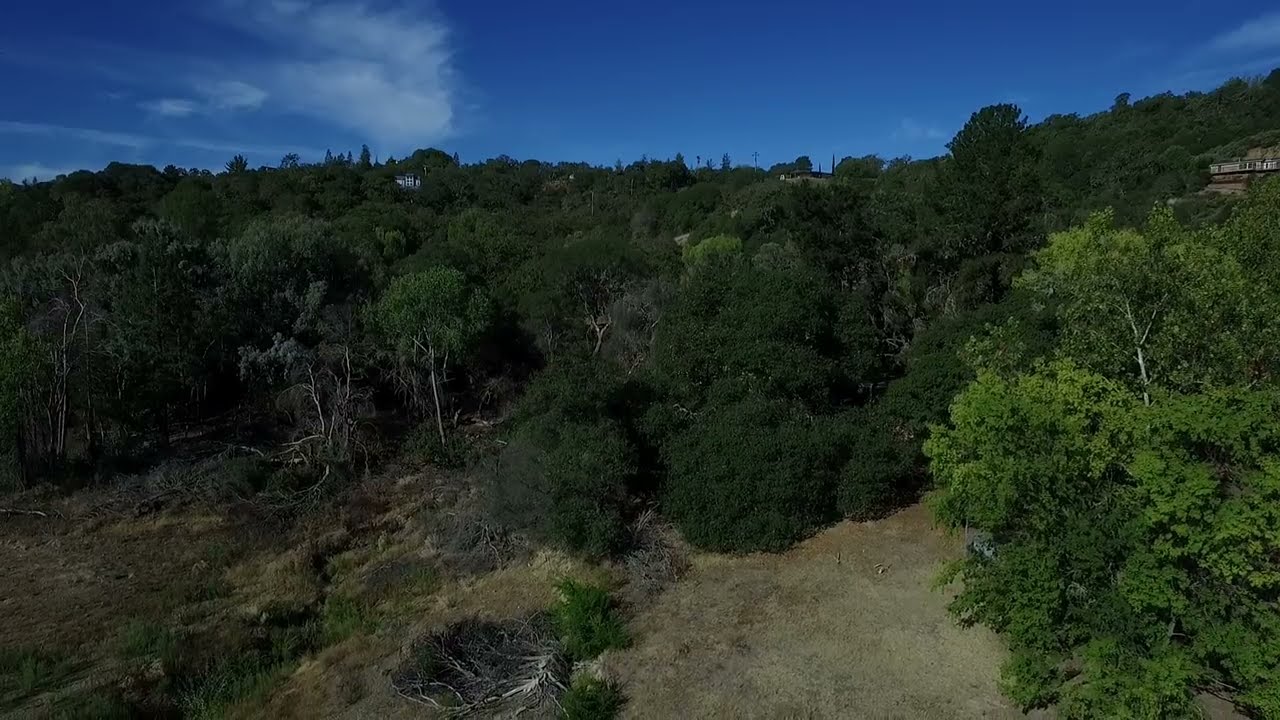The image captures a vast woodland view, taken from a moderately elevated vantage point. The foreground features a dry, grassy area intermixed with dirt and brush, some of which appears to be decaying. Scattered among this terrain are various dead trees and branches, and patches of white bark or tree roots. The woodland itself is dense, dominated by a mix of tall deciduous trees with contrasting light and dark green leaves. The landscape rises gradually to the right, forming a hillside that hosts several structures. Notably, there's a house with a white deck rail in the distant hills to the right, and other smaller buildings partially obscured by the trees and located in clearings within the woodland. On the left side, a tall white building emerges from the forest. The horizon is marked with a blue sky, sparsely decorated with high, wispy clouds, creating a serene backdrop to the expansive forest below.